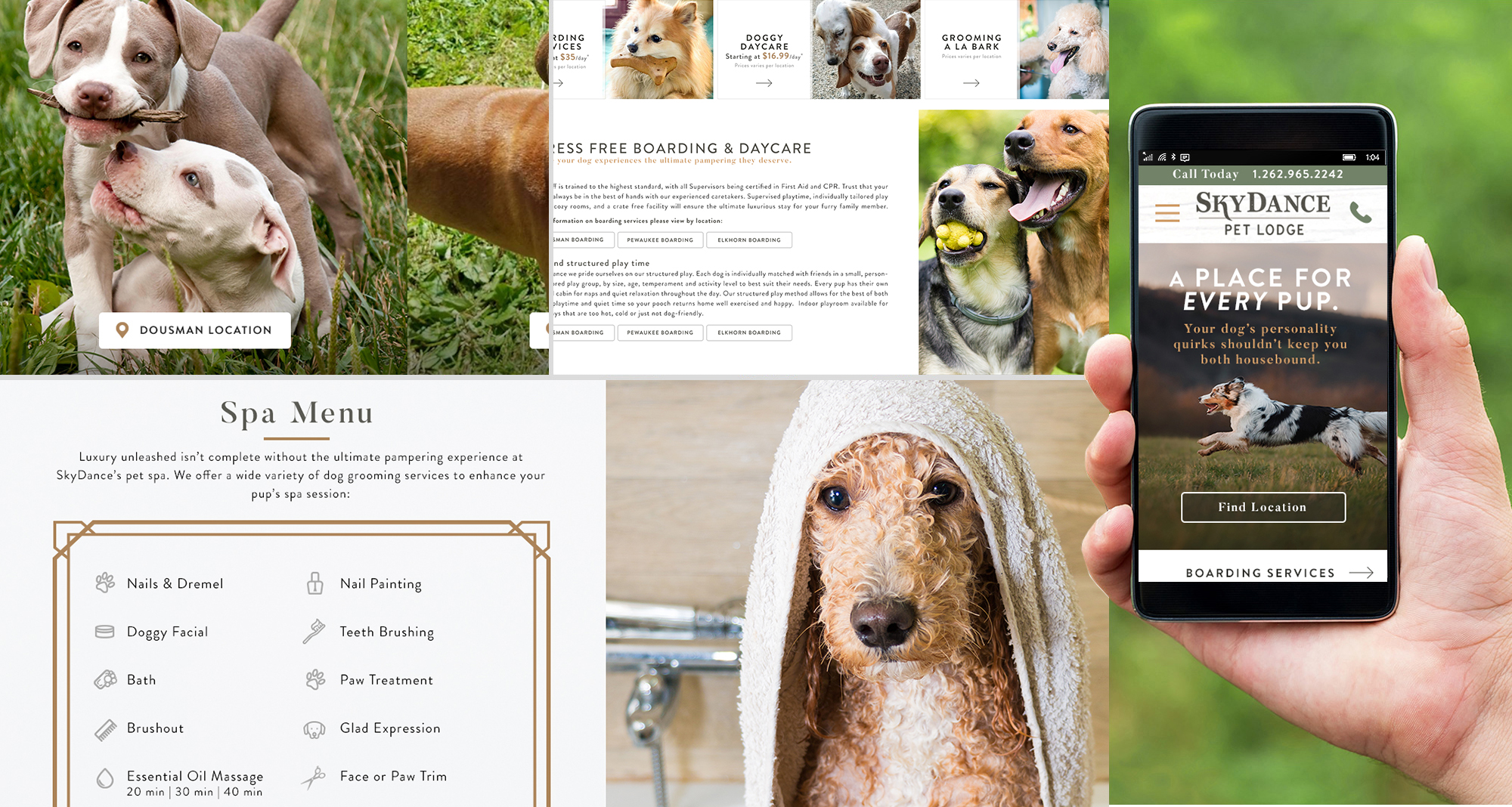The image showcases an advertisement for Skydance Pet Lodge, a dog boarding facility. The central focus is on a person's hand holding a smartphone, with the screen displaying the Skydance Pet Lodge website featuring the tagline "A Place for Every Pup." The top section of the screen shows two adorable puppies playing on the grass, one of them joyfully holding a stick in its mouth. Below this, there's another picture slightly cut off, showing only the body of a dog, adding a quirky touch to the layout.

The website includes a detailed spa menu for dogs, offering services such as nail trimming, doggie facials, baths, brush outs, essential oil massages, nail painting, teeth brushing, paw treatments, and facial or paw trims. 

In the middle section, there seems to be mention of boarding and daycare services, though the exact phrasing isn't fully visible, suggesting it’s a premium rather than a free service. Scattered throughout the advertisement are multiple images of happy dogs in various activities - some are playing with balls, some display cute hairstyles, and others have sticks in their mouths. Among these images, a notably charming picture stands out, featuring a recently bathed dog with a towel draped over its head, encapsulating the comprehensive care provided by Skydance Pet Lodge.